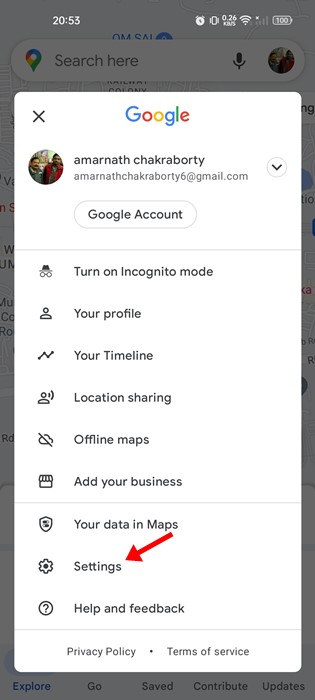"Screenshot of a Smartphone Interface and Google Settings Menu:

The screenshot, captured from a smartphone or tablet, shows the device's status bar depicted in military time at 20:53 in white text. On the right side of the status bar are several icons: a clock, a silhouette of a vibrating smartphone, '0.26 kb/s', a fully-lit Wi-Fi symbol, a cellphone signal icon in gray with a white 'X' above it indicating a missing or damaged SIM card, and a battery icon displaying '100%', though it is transparent with the percentage inside it.

Below the status bar, a pop-up displaying a Google account menu is visible. This includes two Indian men standing close together: one in a gray coat with white accents and another in a red coat with black accents and an undershirt, featured in the top right of the search bar. To the left, there's a black 'X' for closing the menu, and the Google logo, characterized by a multi-colored capital 'G'.

The account menu shows an email address ending with '6@gmail.com' and includes an option in an oval to 'Change account' in black text. Several settings are listed below, each accompanied by icons:
1. Incognito mode: A hat with binoculars, captioned 'Turn incognito on.'
2. Profile: A silhouette of a person, labeled 'Your profile.'
3. Timeline: Represented by a graph.
4. Location Sharing: Depicted with a person emitting sound waves.
5. Offline Maps: An image of a cloud with a slash through it.
6. Add Your Business: Illustrated by a square with a canopy.
7. Your Data in Maps: Shown with a shield with a percentage sign.
8. Settings: Denoted by a gear icon, with a red arrow pointing to it indicating the recommended option for the user to select.
9. Help and Feedback: A circle with a question mark.

At the bottom of this menu are links for 'Privacy Policy' and 'Terms of Service' with dots separating them."